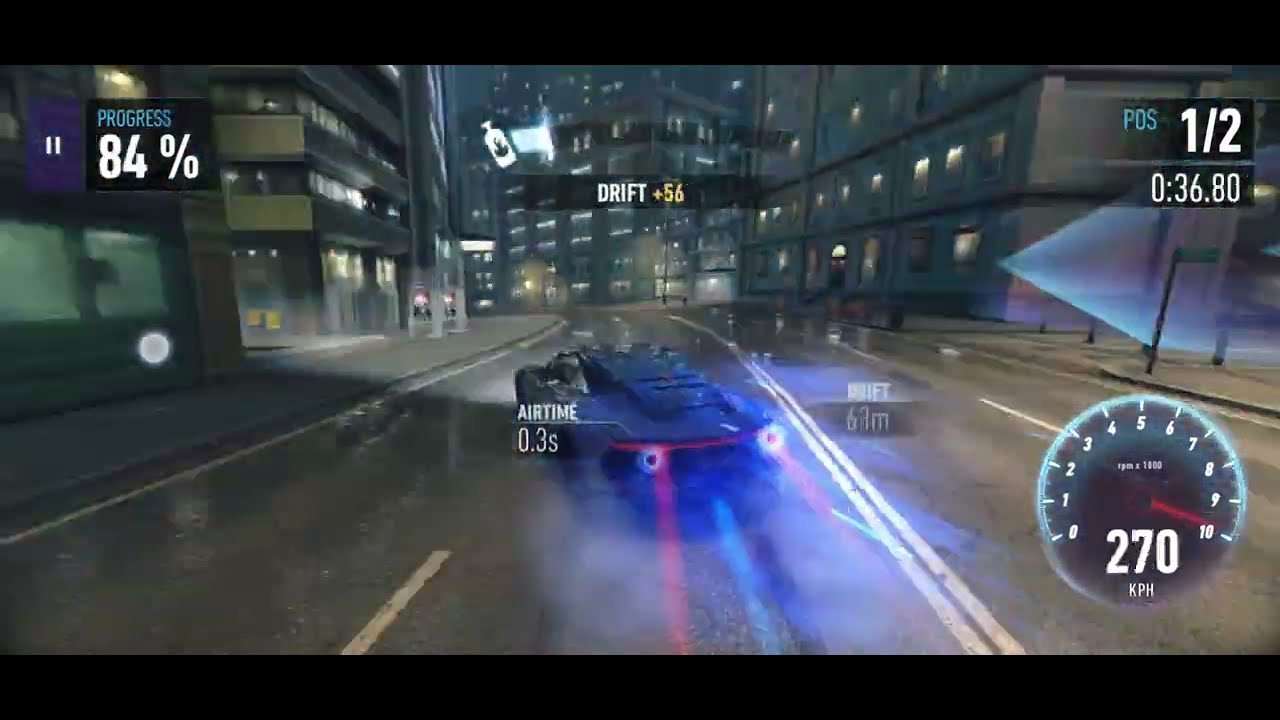This detailed screen grab from a nocturnal, urban racing video game captures an intense moment of high-speed action. The image is framed by black horizontal borders at the top and bottom, timestamping the game as paused at 84% progress. The HUD displays comprehensive data: on the right side, a maxed-out RPM gauge marked from 0 to 10 boasts a speed of 270 kph, surrounded by a red indicator. Nearby, additional statistics include a timer at 0:36.80 and "POS 1/2" in the top-right corner, signaling the player’s top rank. The central focus is a sleek black sports car illuminated by a prominent, continuous red brake light and streaks symbolizing its velocity. Below the vehicle, the text "air time 0.3 seconds" highlights a brief airborne maneuver. The cityscape features lit skyscrapers, storefronts, wide sidewalks, and gleaming reflections off the rain-slick streets, enhancing the intensity as the car tears through a four-lane road, curving left amid this vibrant, rain-soaked metropolis.